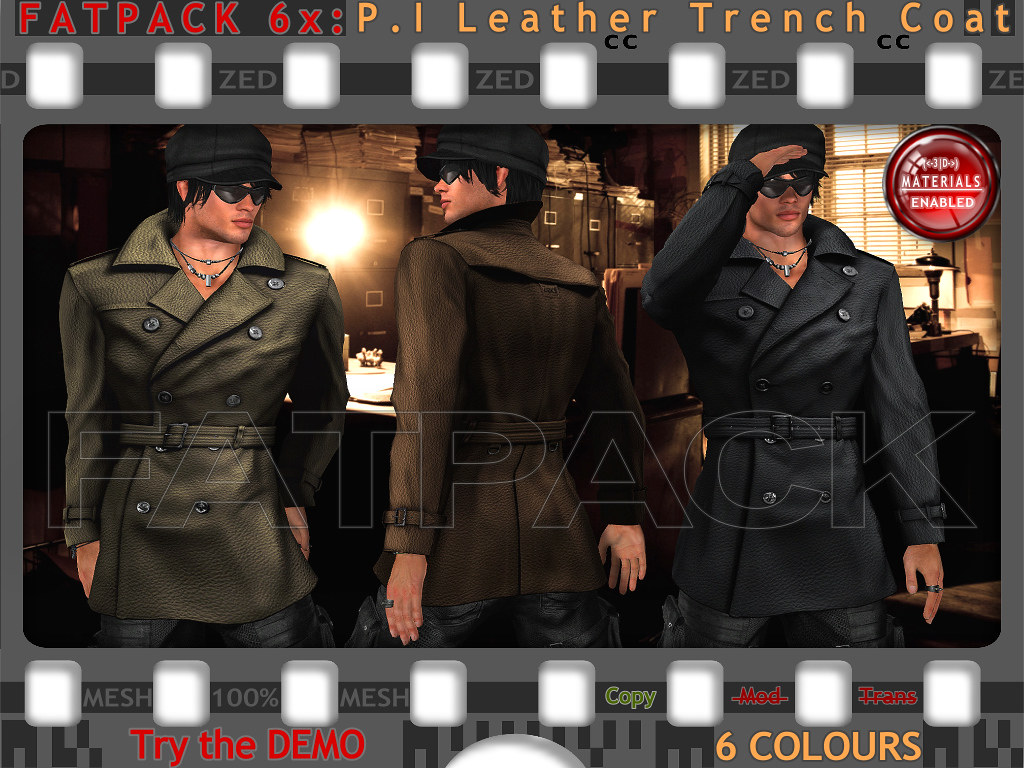This advertisement, styled like a film strip, showcases a computer-generated image of three men modeling hip-length leather trench coats in three different colors: black, brown, and olive green. Each man wears a black hat and sunglasses, with the central figure appearing twice—once from the back and once with his hand shielding his eyes. The ad features a gray border and white squares running across the top and bottom, filled with red and yellow text. Prominently, it reads "Fat Pack 6X: P.I. Leather Trench Coat" in red letters and "Z.E.D." in gray. An eye-catching red button states "Materials Enabled," and at the bottom, "100% Mesh Copy Mod Trans" is displayed. Yellow text highlights "Six colors," and red text at the very bottom urges viewers to "Try the Demo."